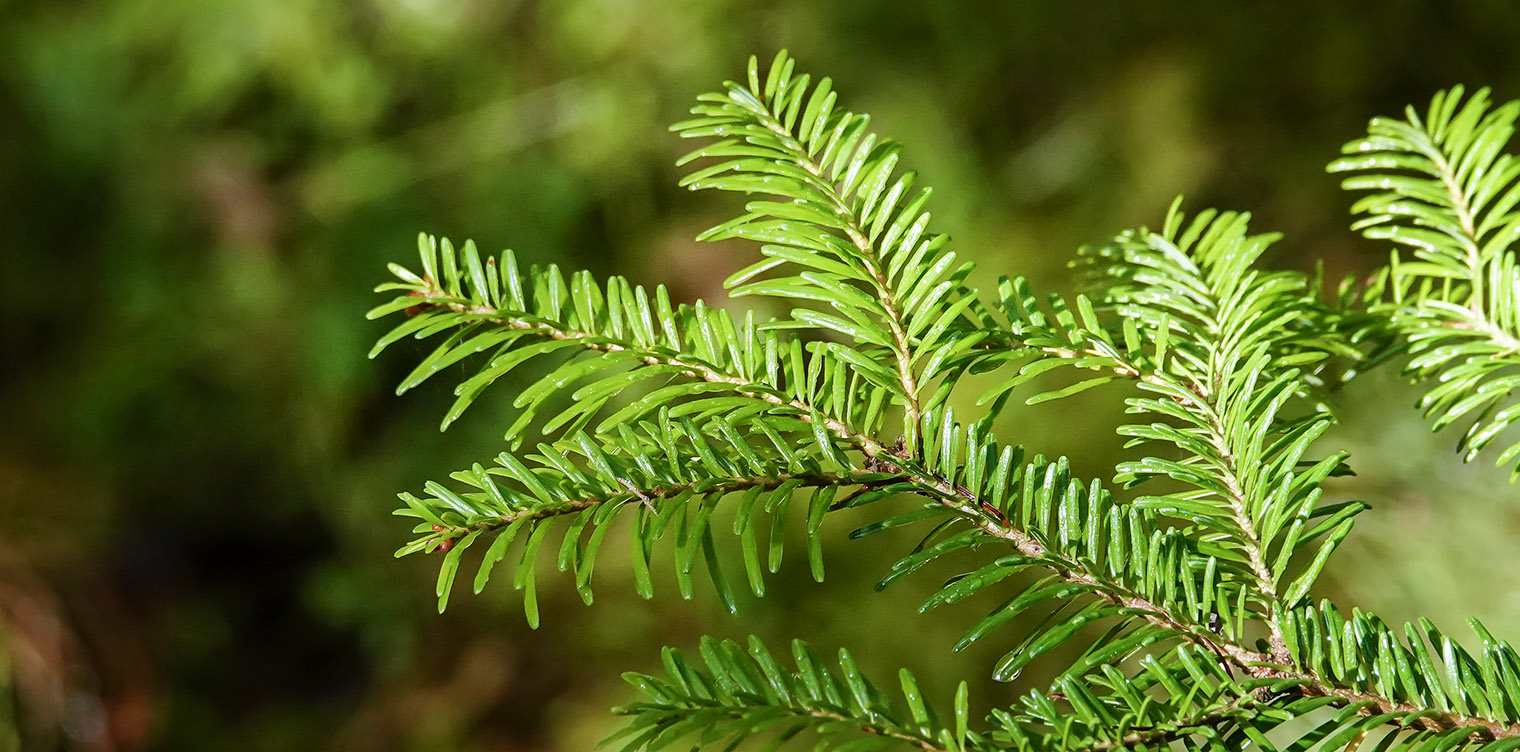The photograph features a close-up of a single branch from a plant that resembles a Christmas tree or a pine tree, though it may also be a fern. The branch is detailed and highly textured with multiple green, straight, and shiny needle-like leaves extending from it. The branch itself is brown, providing a stark contrast to the vibrant green leaves. The composition of the image thoroughly focuses on this one branch, capturing its intricate structure, with individual sub-branches or "twigs" visible, numbering around ten or more on various sides. The background is out of focus and blurry, filled with hues of green and brown, suggesting a forest or dense foliage behind the branch. Sunlight filters through the scene, illuminating the top half of the branch and casting light throughout the image, enhancing the vividness of the green leaves. The photograph accentuates the minute details and natural beauty of this specific branch against a soft, sunlit backdrop.